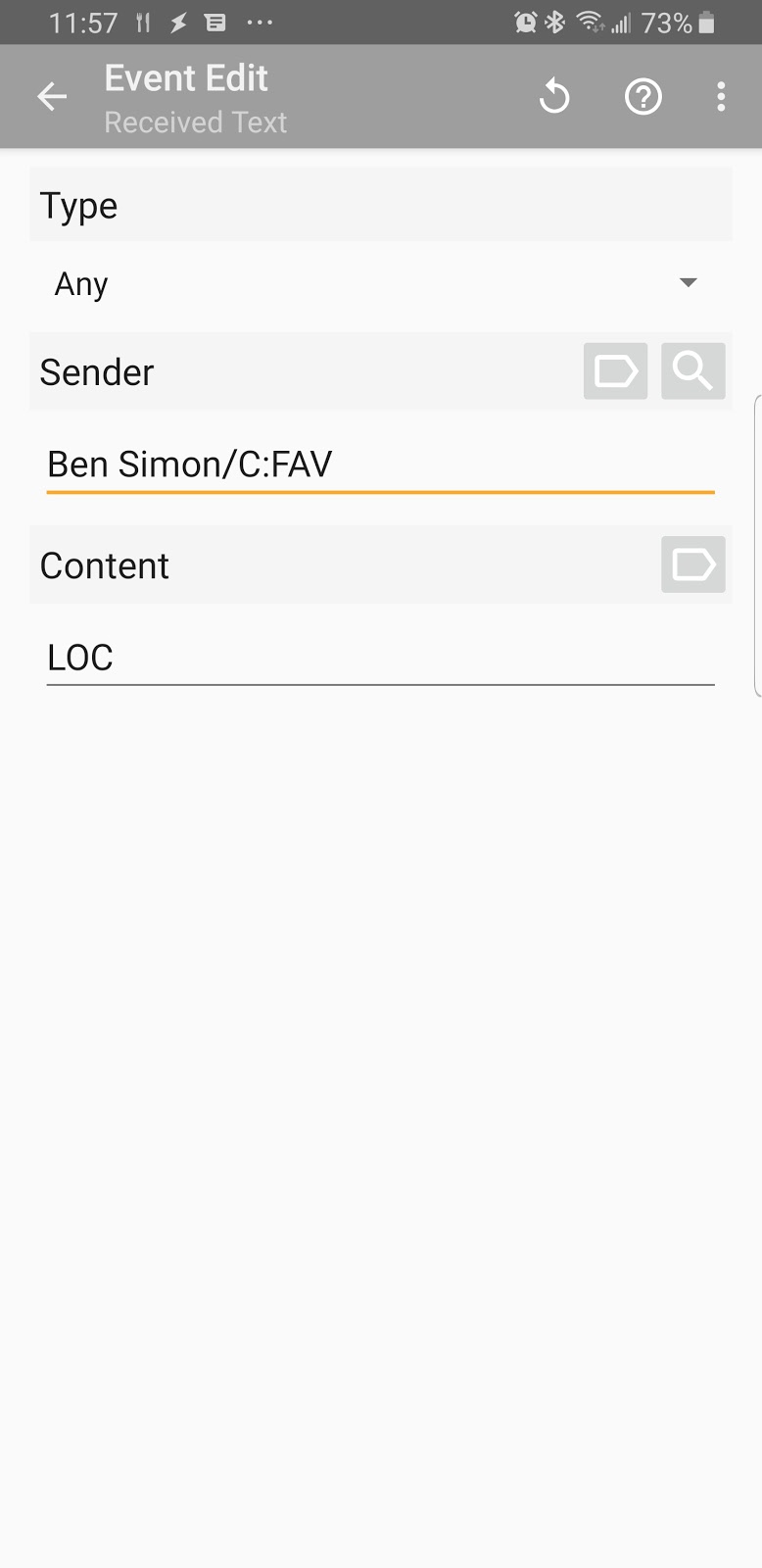The screenshot, taken from either a tablet or smartphone, captures a detailed interface. At the top, encased in a black bezel, the display time reads "1157" in military format. The status icons include two exclamation marks, a lightning bolt, and a chat notification icon with three ellipses. On the right, an alarm clock icon is followed by Bluetooth, full WiFi, and nearly full cellular signal bars. The battery level is indicated at 73%.

Below the status bar, a large dark grey rectangle displays "Event Edit" in white text with a white arrow pointing left. Beneath this header, lighter grey text reads "Received Text". To the right, a refresh arrow (curved like a 'C'), a question mark inside a circle (indicating help or information), and another set of three ellipses are aligned.

The section beneath contains a mid-grey rectangle with various lighter bands. On the left, cascading black text reads "Type Any Sender Ben Simon \c.. FAV" (with "FAV" in all caps). Following this, the terms "Content" and "Lock" are seen. Adjacent to "Content" and "Sender" are arrows and a magnifying glass icon, while next to "Any", there is a black drop-down arrow. "Ben" is underscored with an orange line and a grey line appears beneath "Lock".